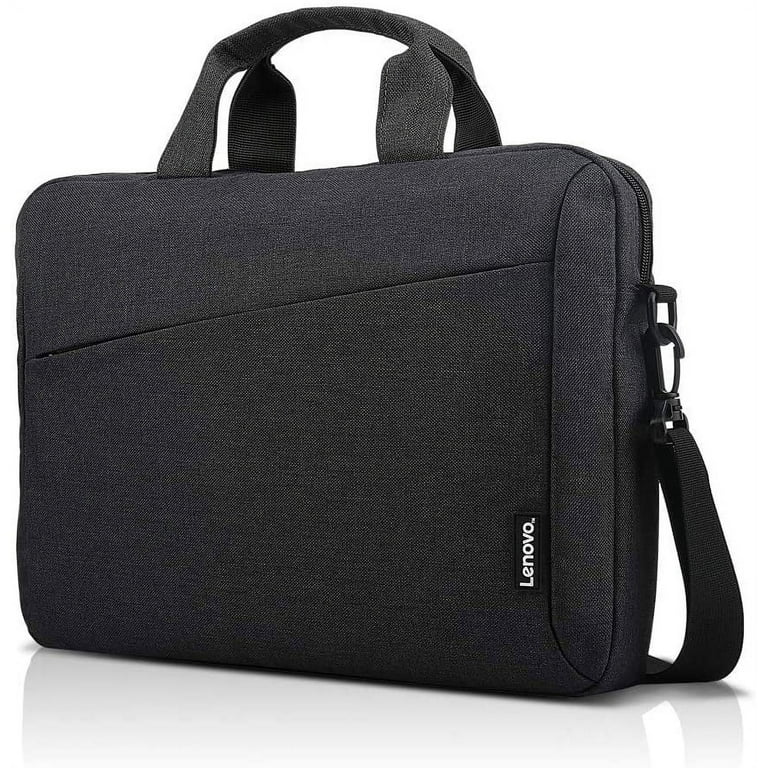The image depicts a Lenovo laptop bag made of charcoal gray, tightly woven canvas material. The bag is rectangular in shape and features both a set of two darker gray fabric handles arching over the top and a long, black shoulder strap that attaches at a hook on the side, draping down and behind the bag, touching the floor. There is a zipper closure that runs from the far right side of the bag up and around the top to the left. Additionally, a diagonal zippered pocket runs from the top right to the middle left on the front side of the bag. A small white fabric tag with black background and white lettering displaying the Lenovo brand is located on the bottom right corner along the seam. The bag is presented against a white background, with its shadow visible, highlighting its sleek and functional design.